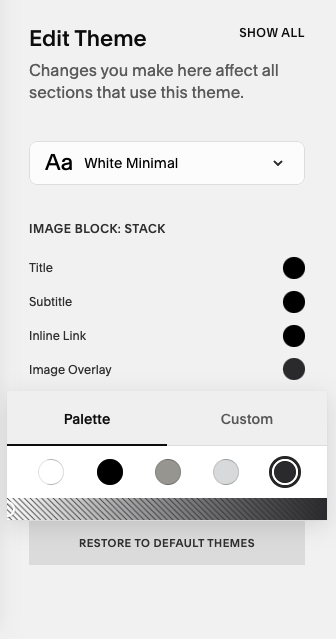Captured in this image is a user interface design screen focusing on theme editing options. The background displays a lilac color scheme typical of mobile phones. On the right side of the screen, there's a dropdown menu currently set to a font style labeled 'White Minimal' denoted by an icon of a capital 'A' alongside a lowercase 'a'. 

Moving on, there are four specific customization areas titled: 'Title,' 'Subtitle,' 'Inline Link,' and 'Image Overlay,' each accompanied by color settings. The 'Title,' 'Subtitle,' and 'Inline Link' options are all set to black. The 'Image Overlay' appears to be a lighter shade, almost gray but leaning towards black.

Below these options, there is a 'Palette' section which is active. It offers a selection of color swatches including white, black, gray, light gray, and a slightly darker gray circled for emphasis. To the right of the palette, there's an option for 'Custom' color settings. At the very bottom of the interface, there's a button labeled 'Restore to Default Themes' to revert any changes.